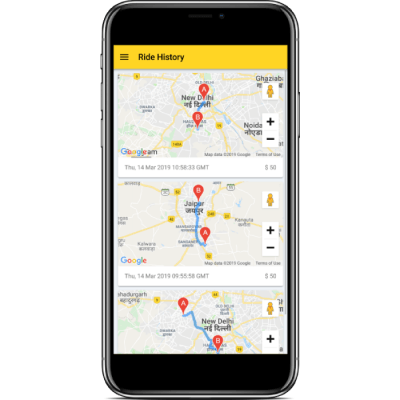The image features a black iPhone with silver or gray edges, displaying a detailed simulation of an app interface. The phone's screen prominently shows a yellow banner at the top with the black-font text "Ride History." To the left of this title is a menu icon, depicted as three horizontal lines stacked vertically.

Below the banner are three sections depicting maps sourced from Google Maps, each illustrating the route of a journey. These routes are marked by red pins labeled "A" and "B" with white lettering, connected by blue lines indicating the travel path. The backgrounds of these maps are primarily a light tan-gray shade, with yellow lines delineating major roads and highways.

In the bottom left-hand corner of each map section, the Google logo is visible. Additionally, below each map, there is a banner displaying details such as the date, time, and possibly the cost of the ride, although the third map's banner is partially cut off and not fully visible. The maps also highlight various cities and feature zoom in/out buttons, along with an icon of a yellow purse on the right-hand side of each map.